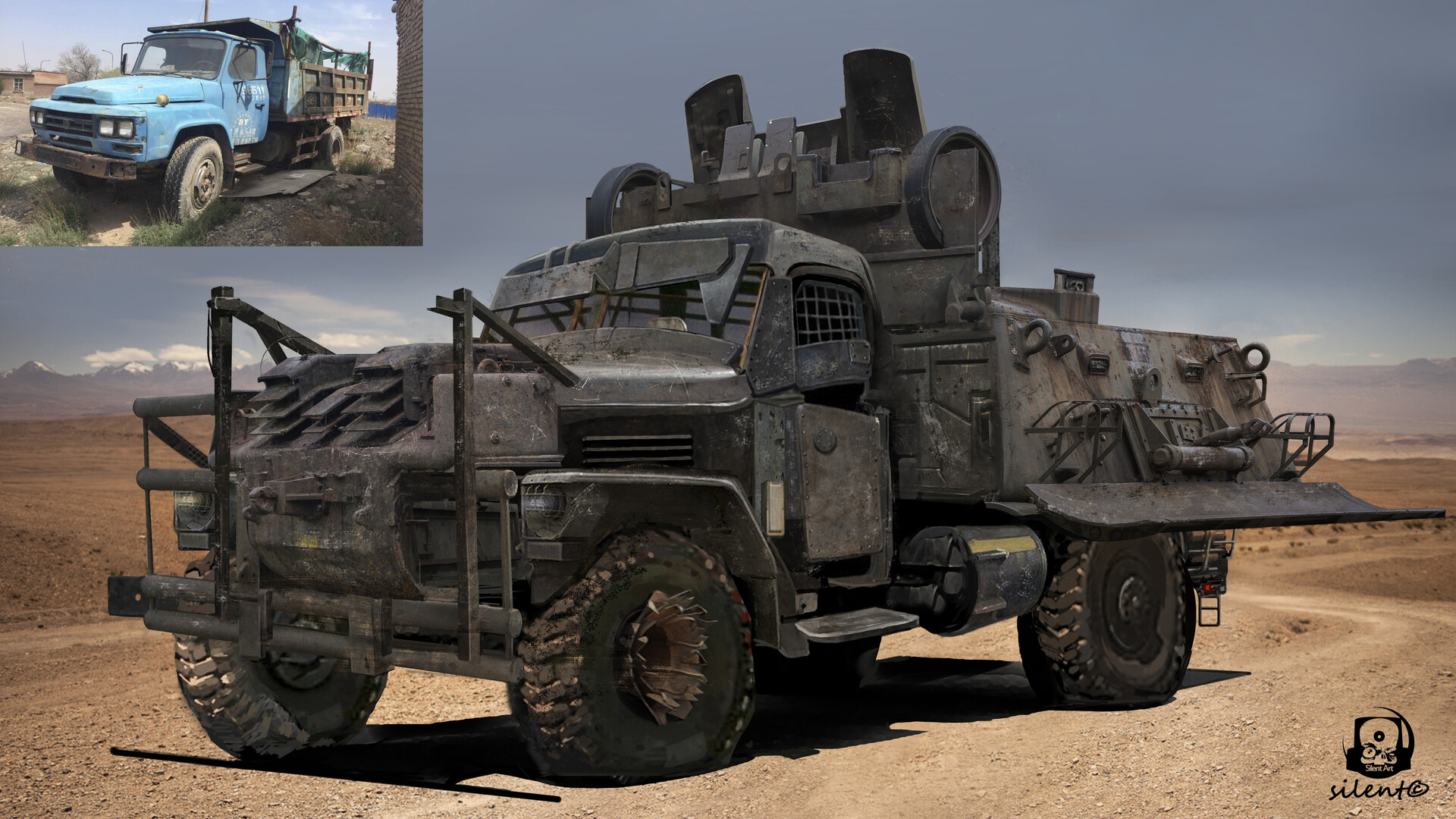The image features a detailed 3D rendering of a militarized vehicle set against a desert environment. Dominating the scene is a black, armored truck equipped with large spiked wheels, metal reinforcement bars on the front, and utility hooks and machinery on the back. The vehicle also has bars on the windows, a tool holder, a shovel lift, and two lights mounted on the top, evoking a rugged, post-apocalyptic style reminiscent of "Mad Max." In the upper left-hand corner, there is a smaller inset image of the truck that served as the inspiration for this rendering. This smaller picture depicts a blue vintage civilian work truck from the 70s, distinguished by its white side lettering, green tarp-covered carrier on the back, and its setting in a bright daytime desert scene with blue skies and a mountain in the background. This realistically dirtied old truck starkly contrasts with the sophisticated and heavily armored appearance of the rendered vehicle. The rendering is a creation by an artist named Silent, showcasing a blend of old and new, civilian and military elements.